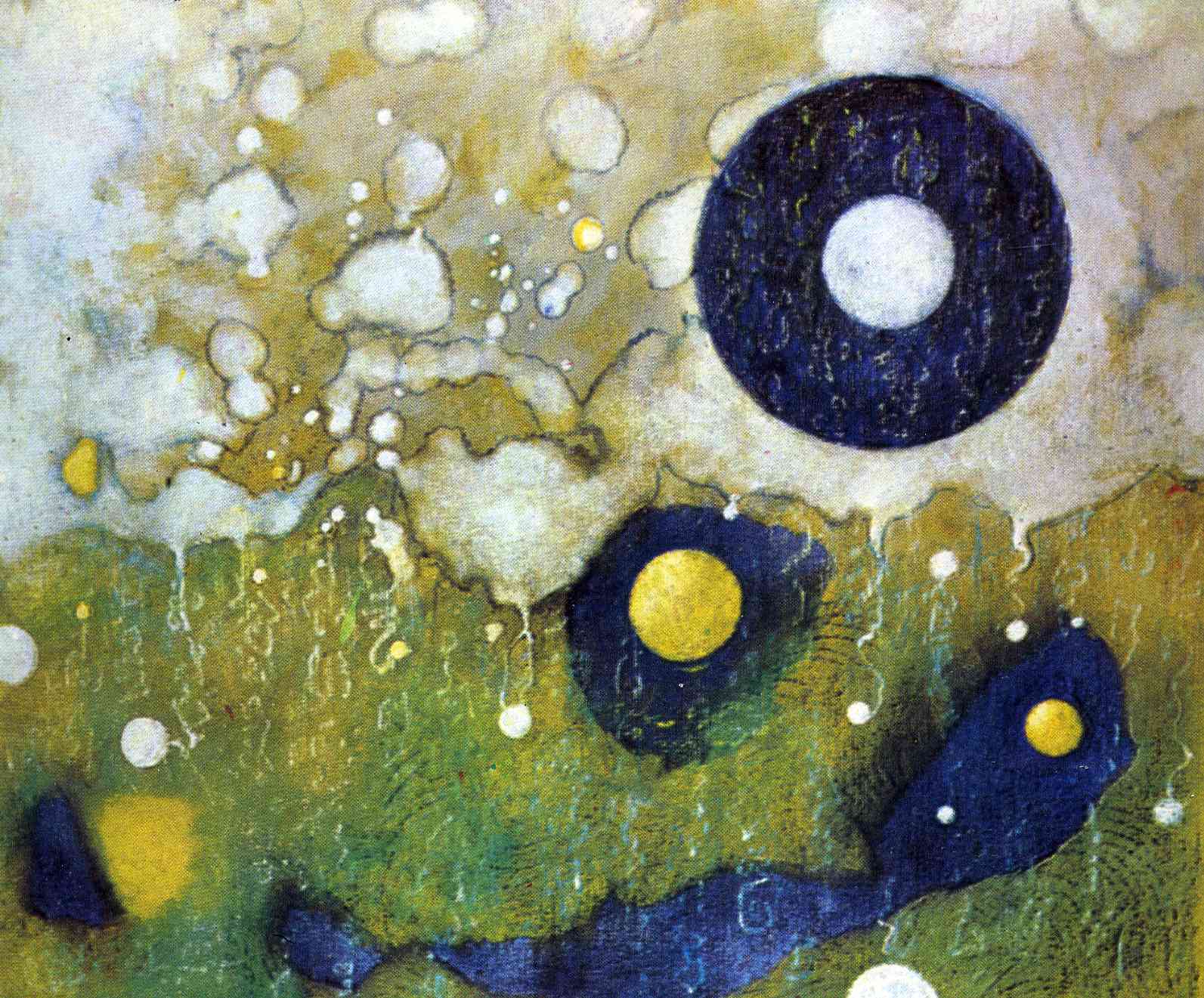This painted image features a surreal landscape composed of various shapes and colors. At the bottom, a grassy plane painted in green serves as the foundation. Scattered across this grassy base are peculiar splotches of purple and black. Above this area, the painting transforms into an abstract scene where elements of nature and whimsical forms intersect.

Dominating the upper right section is a large blue donut shape, characterized by a hollow center and framed by streaks of variegated colors. Surrounding this form is an expanse filled with white foam, evoking the appearance of soap suds. These suds extend across the backdrop, creating formations reminiscent of clouds and even a poodle shape, adding a playful touch to the sky.

Towards the center-left area, there's another circle, although not quite complete, featuring a striking yellow dot at its core. This circle appears as if it has melted away, leaving an unfinished blue border. Moving downward, a dark blue ribbon-like shape starts from the bottom right and meanders towards the left, embedded with a large yellow dot and accompanied by patches of navy blue and smudges of yellow paint.

Overall, the painting captures a mesmerizing blend of shapes and colors, from dripping white droplets to smears of blue and yellow, all harmoniously coexisting to form an imaginative and detailed visual experience.